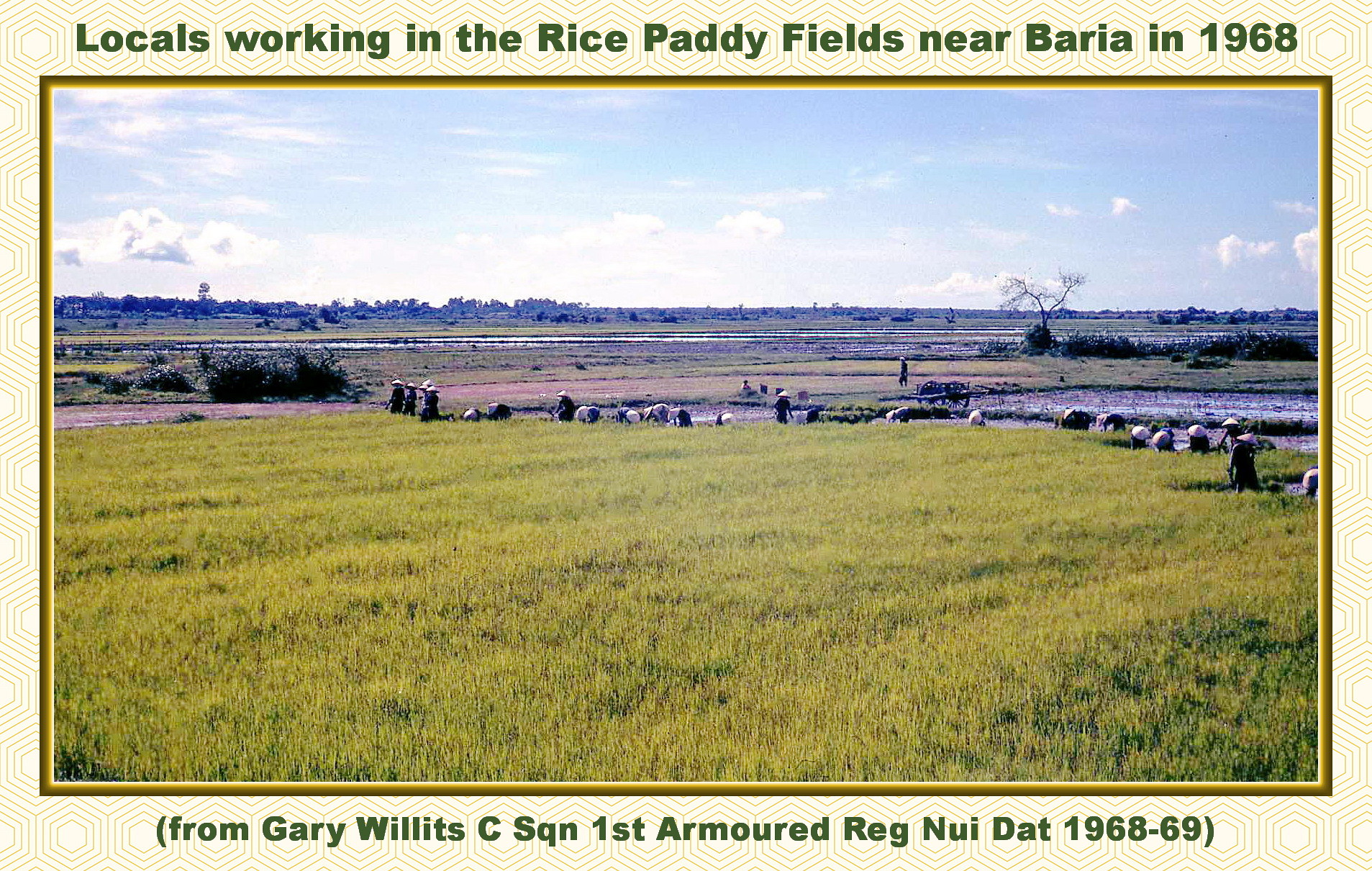This image, taken in 1968, depicts locals working diligently in the rice paddy fields of Erebaria, Vietnam. It captures roughly 30 individuals, clad in traditional conical straw hats, bending over and carrying sacks as they tend to their crops. The scene is set under a clear blue sky dotted with distant clouds, with the sun high, casting bright light over the expansive field. The muddy depression areas are framed by very tall grass, characteristic of rice fields, which is essential, though it appears sparse. In the far distance, trees and a large lagoon form part of the picturesque agricultural landscape. The photograph is bordered with a beige trim accentuated by a thin mustard-colored line. Originating from Squadron 1st, Armored Regiment, Nui Dat, during the Vietnam War, the image is noted to be from the collection of Brinkeri Willis C/Gary Willett, capturing a significant historical and cultural moment.